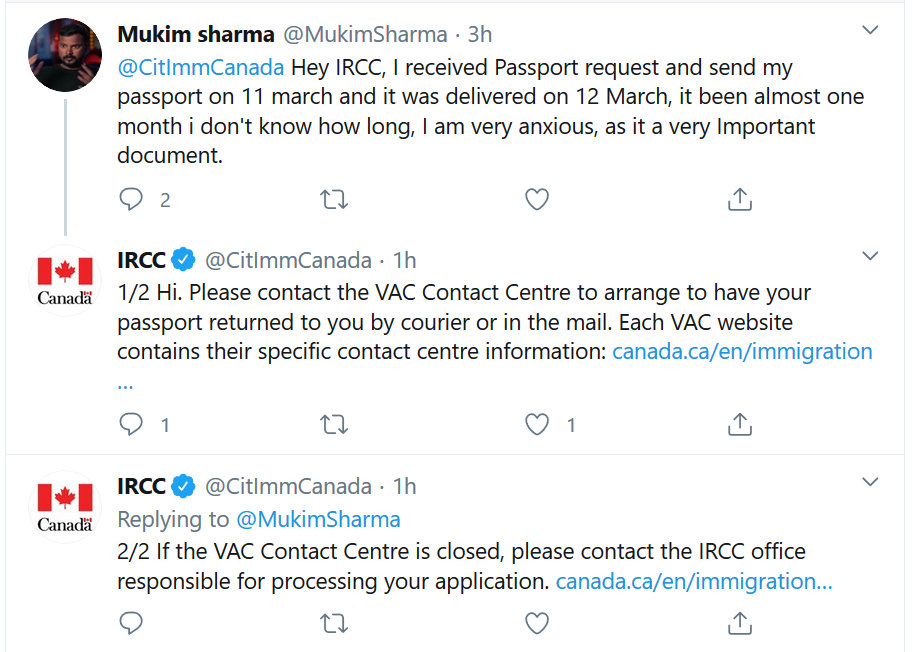The screenshot captures a conversation on Twitter involving a tweet by Mukum Sharma and two replies from IRCC, the Immigration, Refugees, and Citizenship Canada. Mukum Sharma’s tweet, posted three hours ago, appears to be directed at IRCC (@IRCC) seeking assistance with an issue related to passport retrieval. The replies from the verified IRCC account, which has a Canada flag as the profile picture and the username "Canada" in black text, are split into two parts. 

In the first part of the response, IRCC advises Mukum to contact the VAC (Visa Application Center) contact center to arrange the return of his passport either by courier or mail. They mention that each VAC website contains specific contact information. 

The second part of the tweet informs Mukum that if the VAC contact center is closed, he should contact the IRCC office responsible for processing his application. The URL "Canada.caenimmigration" is also provided to guide users seeking more information.